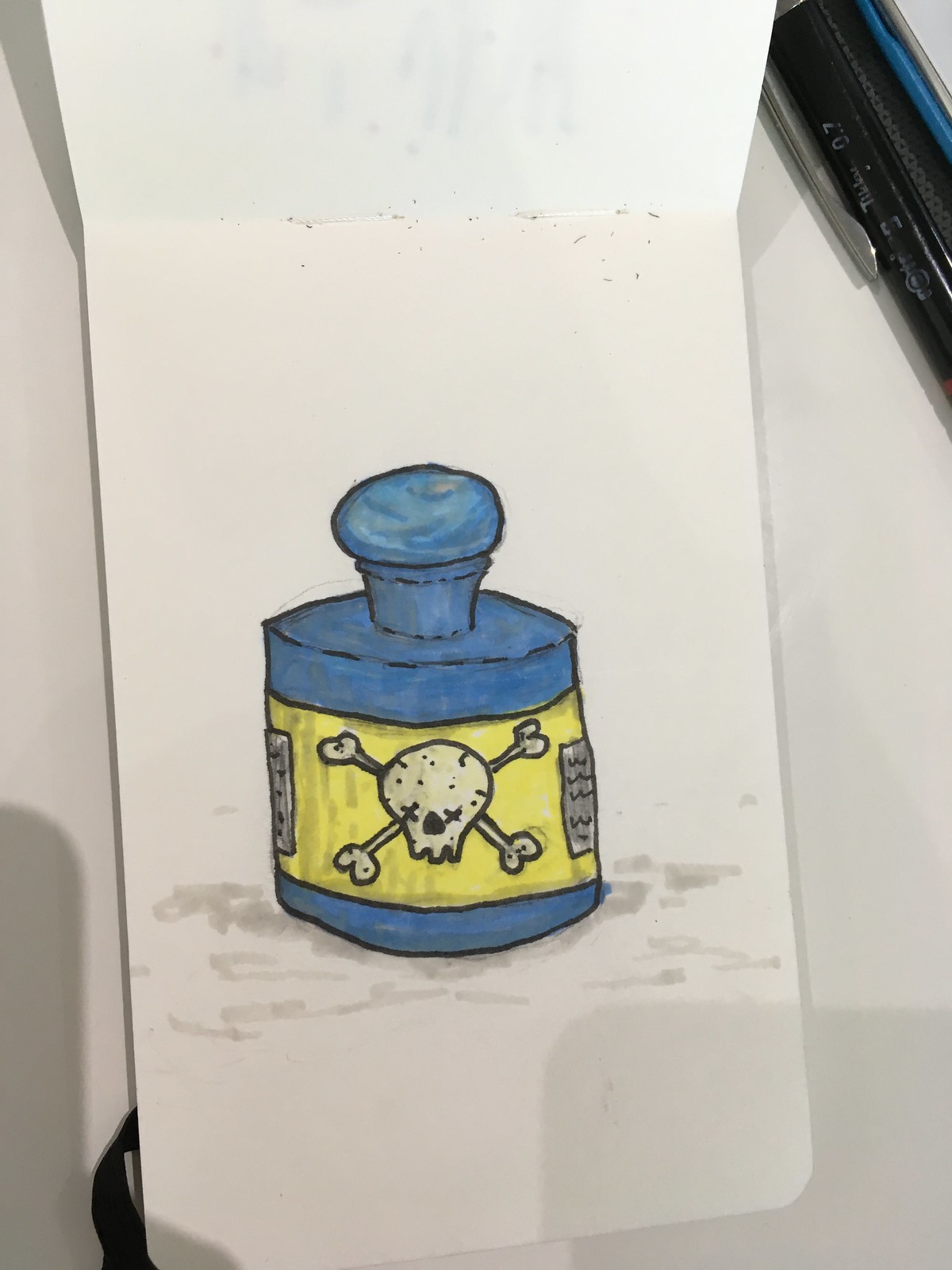The image showcases a child's hand-drawn depiction of a bottle of poison, captured from above on a white piece of paper that extends slightly out of the notebook frame at the top. The drawing is relatively small, comparable in size to a post-it note, as indicated by a pen lying nearby for scale. The blue, round bottle features a short neck and a circular lid, rendered in what appears to be blue magic marker. A yellow horizontal label wraps around its middle, adorned with a childishly drawn tan skull and crossbones. The skull has simple X's for eyes and a black gap representing the nasal cavity. Surrounding the label, there are small, illegible drawn panels that resemble instructions. Two pens can be seen at the upper right corner of the photograph, adding to the sense of scale and placement. Beneath the bottle, light gray dashes suggest a surface beneath it, completing the cartoonish portrayal.